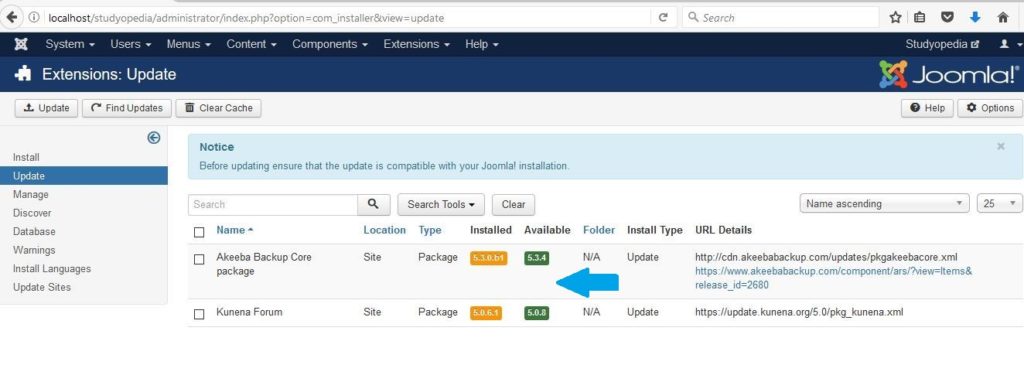Screenshot of a Joomla Website Backend

This screenshot captures the backend interface of a Joomla-powered website. At the top of the image, there is a URL displaying 'localhost,' indicating that the site is likely running on a local server. Right below the URL, the website's top navigation bar is visible in a dark blue shade. This bar hosts seven menu items, each accompanied by a downward-facing arrow icon, signifying that they are drop-down menus. The menu items include Systems, Users, Menus, Content, Components, Extensions, and Help.

Positioned on the far right of this dark blue navigation bar is the Joomla logo, comprising four interlinked chain links in green, yellow, blue, and red, alongside the text 'Joomla.' Just below this bar, on the left side, a distinct white puzzle piece icon precedes the text 'Extensions Update,' signaling the section currently being viewed or highlighted.

Occupying the left side of the screenshot is a gray sidebar, offering additional navigation and options pertinent to the website management. On the right side, a light blue notice stands out, likely containing important information or an alert for the site administrator. The image encapsulates the organized and detailed layout typical of Joomla's administrative interface, facilitating ease of use for website managers.